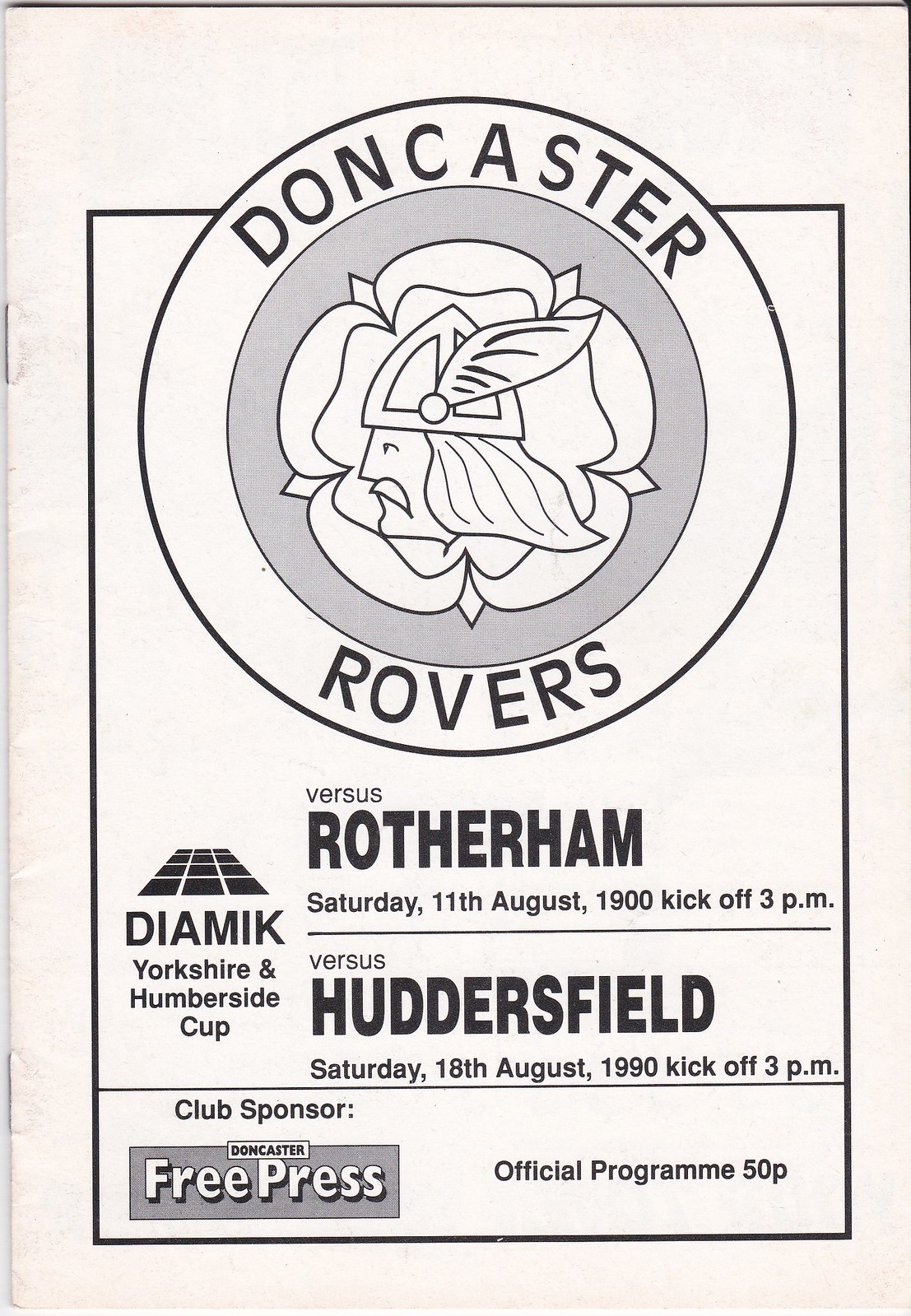This image depicts an older soccer program primarily featuring a white background with black text and gray accents. At the center top is a large circular logo that reads "Doncaster Rovers," with "Doncaster" above and "Rovers" below. This logo contains an abstract depiction of a Viking, characterized by a helmet with long hair and a feather, looking to the left. Below the logo are details of two matches: "Versus Rotherham, Saturday, 11th August, 1900, kickoff 3 p.m." and "Versus Huddersfield, Saturday, 18th August, 1990, kickoff 3 p.m." On the left, the text reads "Diamick, Yorkshire and Humber side club." At the bottom, it states "Club Sponsor, Doncaster Free Press," and in the bottom right corner, it is labeled "Official Program, 50p."